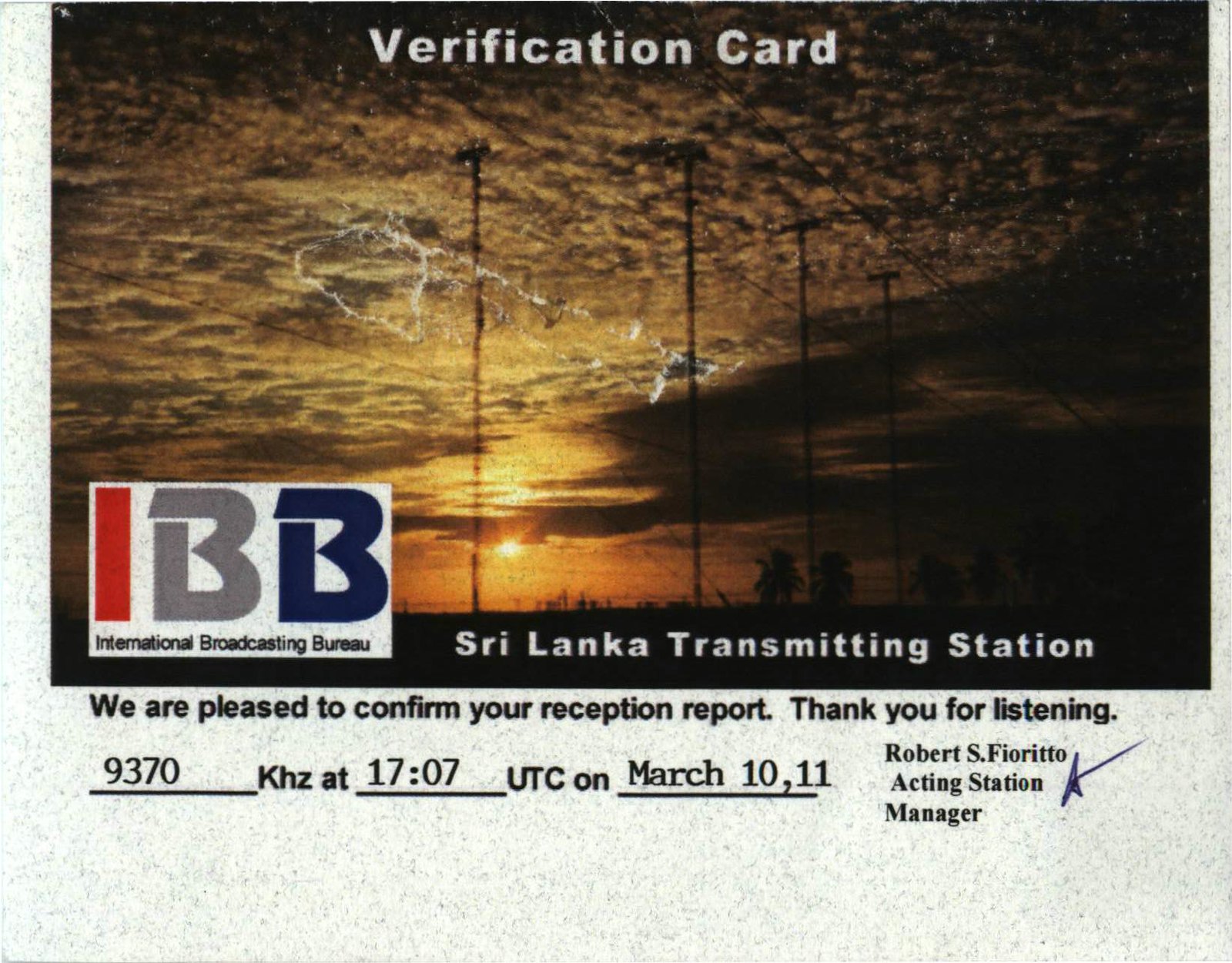The image depicts a verification card from the International Broadcasting Bureau (IBB) for the Sri Lanka Transmission Station. The card features a photograph of a cloudy, dark golden-brown sky with streaks resembling lightning. Tall electrical poles and silhouettes of trees are visible in the distance against a speckled grey-white background. At the top, the card prominently displays in white letters "Verification Card" and "Sri Lanka Transmitting Station," accompanied by the IBB logo, where the I is red, the first B is gray, and the second B is blue, enclosed in a white box. Below the photograph, the text reads, "We are pleased to confirm your reception report. Thank you for listening. 9370 kilohertz at 1707 UTC on March 10th and 11th. Robert S. Fiorito, Acting Station Manager," followed by his signature. The card encompasses various colors, including gray, black, red, blue, white, yellow, and orange, and appears to be styled as a postcard issued to a radio station listener.